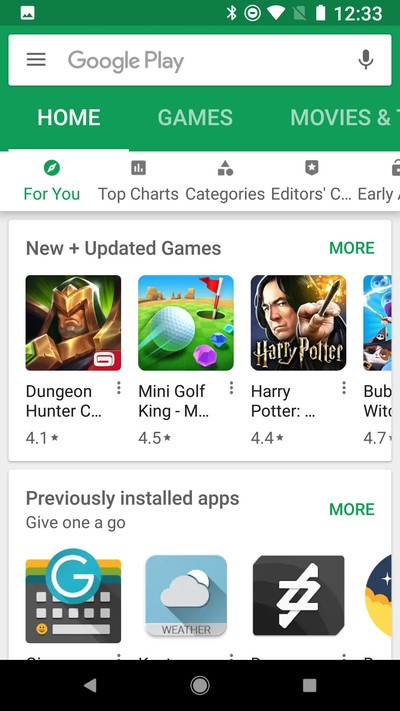This screenshot captures the Google Play Store homepage on an Android phone, showcasing various details and app suggestions. The status indicators at the top reveal that Bluetooth is enabled, the device is connected to Wi-Fi, the battery is fully charged, and the time is 12:33. On this screen, the Google Play search bar stands prominently at the top, featuring a microphone icon for voice search on the right side and three vertical bars on the left.

Currently, the "Home" tab is active, specifically showing the "For You" section. The main focus is on the "New and Updated Games" category, with a visible option to explore more. In this category, three games are highlighted:

1. **Dungeon Hunter**: Rated 4.1 stars, it features an animated character adorned in gold headgear and a breastplate, wearing an intense, angry expression.
2. **Mini Golf King**: Depicts an animated golf ball about to enter a hole, surrounded by jewels and rain of pink balloons.
3. **Harry Potter: Hogwarts Mystery**: Showcases an image of Severus Snape, a character from the Harry Potter series, holding a wand, with the title "Harry Potter" displayed below.

Beneath the "New and Updated Games" section, there's a "Previously Installed Apps" section labeled "Give Me a Go," although specific app details are obscured, showing only partial images.